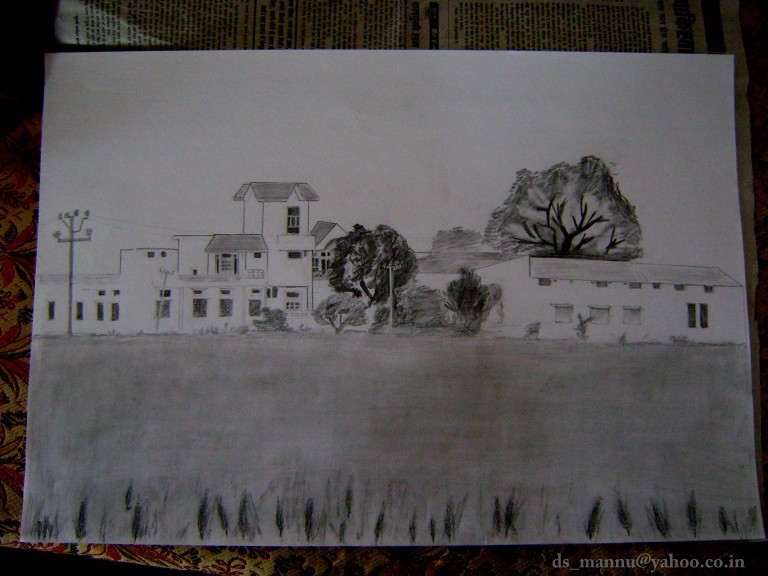This detailed black and white drawing, rendered on a white sheet of paper, captures an outdoor scene. Prominently featured in the composition are several buildings, creating an urban landscape. In the foreground, on the left side, an electrical pole with wires stretches across the canvas, adding a touch of realism and intricacy. At the bottom of the drawing, various plants are depicted, sprouting and encroaching into the scene, providing a contrast to the rigid structures above. The artist's signature, "ds_mannu at yahoo.co.in," is inscribed in white in the bottom right corner, adding a personalized touch to this meticulously detailed work of art.